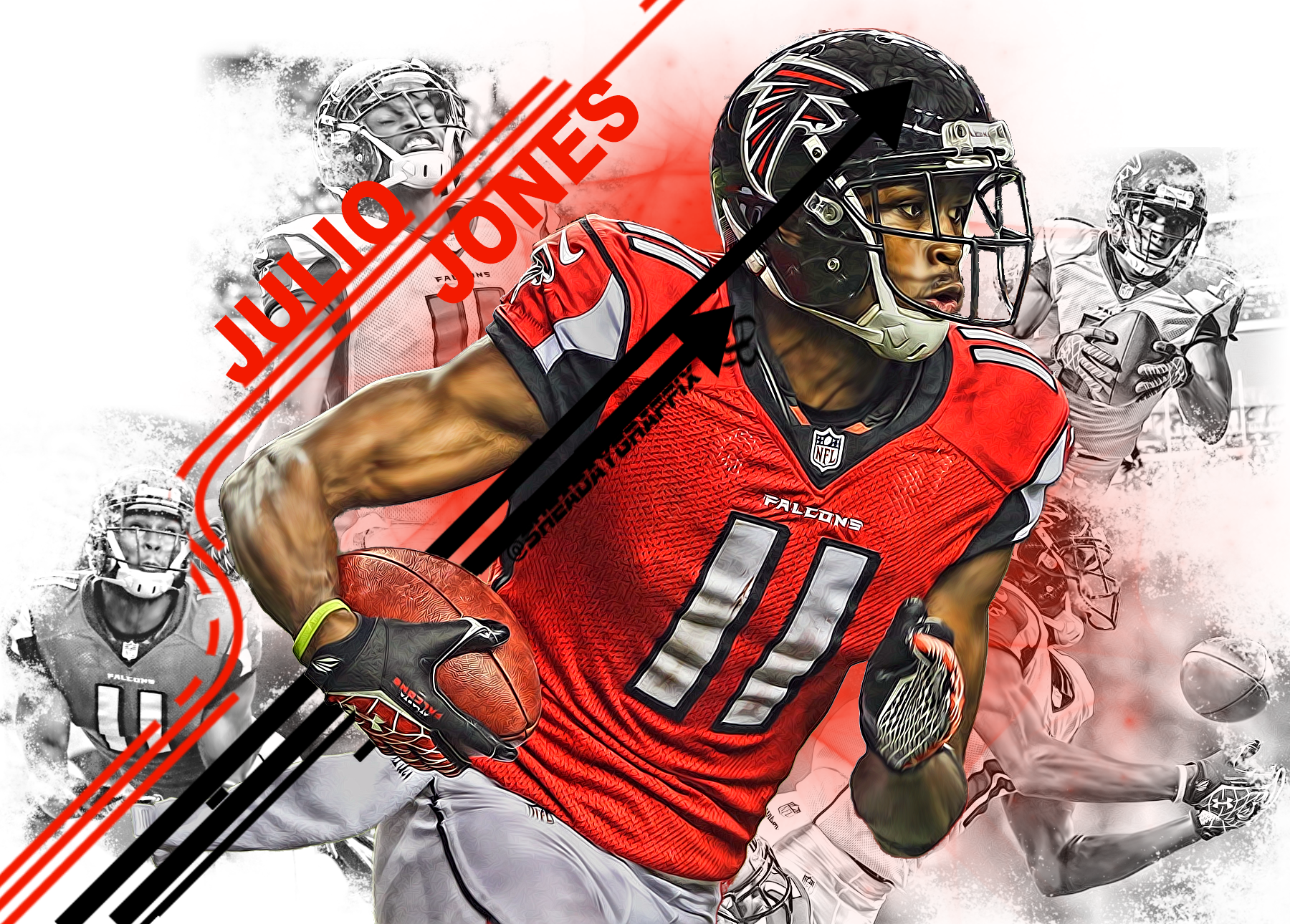The image features an Atlanta Falcons football player, Julio Jones, prominently in the center, captured in the midst of an action-packed run towards the right. He wears a black Atlanta Falcons helmet emblazoned with the team's falcon logo, and a dynamic red jersey with white and black accents. The number '11' stands out in white on his chest and shoulders. The V-neck of his jersey meets at his neck, marked with the NFL logo. Jones's muscular right arm cradles a football, adorned with a black glove featuring red and white designs, and a yellow wristband. His left hand, also gloved, reaches out in front of him. His white football pants extend off the bottom of the image, and the background features vibrant graphic elements.

A series of black and red lines emanate from the bottom left corner, sweeping up and right, culminating in arrowheads. The red lines then zigzag up, left, and right again. The name "Julio Jones" is inscribed in red above and below these lines. Complementing the primary image, black-and-white illustrations of Jones in various action poses fill the upper left, lower left, upper right, and lower right corners, blending seamlessly with the light background to create a dynamic and energetic poster-like composition.